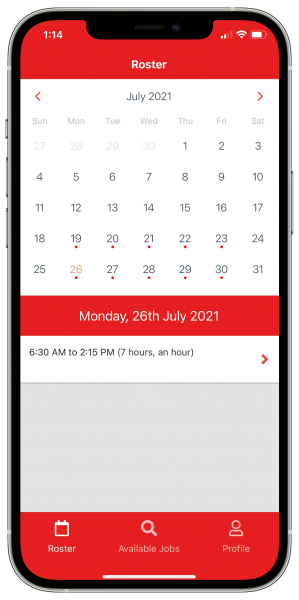This detailed image depicts a high-fidelity mock-up of a smartphone displaying a calendar app interface. The phone's design includes a prominent camera at the top, a sleek metal frame, and responsive side buttons. At the top of the screen, in a red status bar, the time is displayed as 1:14 PM, accompanied by robust signal strength indicating 204 signal bars, full Wi-Fi connectivity, and a battery level at approximately 80%.

The main screen showcases a monthly calendar for July 2021, against a clean white background. The layout starts from Thursday the 1st and concludes on Saturday the 31st, organized into a total of five weeks. Noteworthy are the dates 19th through 23rd and 26th through 30th, marked with red dots underneath, denoting special events or reminders. Additionally, the date 26th is highlighted with red text indicating it as the selected or current day. This is further confirmed by a red panel directly below the calendar stating, "Monday, 26th of July, 2021".

Below this, another white panel details a scheduled event, reading "6.30 a.m. to 2.15 p.m., seven hours," with a red arrow for additional options or actions. The screen's gentle drop shadow effect adds a subtle depth to the interface.

Near the bottom of the screen, just above the red-colored final menu bar, a light gray panel houses user interaction options. The menu bar itself contains four icons: a calendar labeled "roster," a magnifying glass indicating "available jobs," and a generic profile icon with the label "profile." This well-organized and visually appealing mock-up efficiently combines functionality with design elements for a seamless user experience.